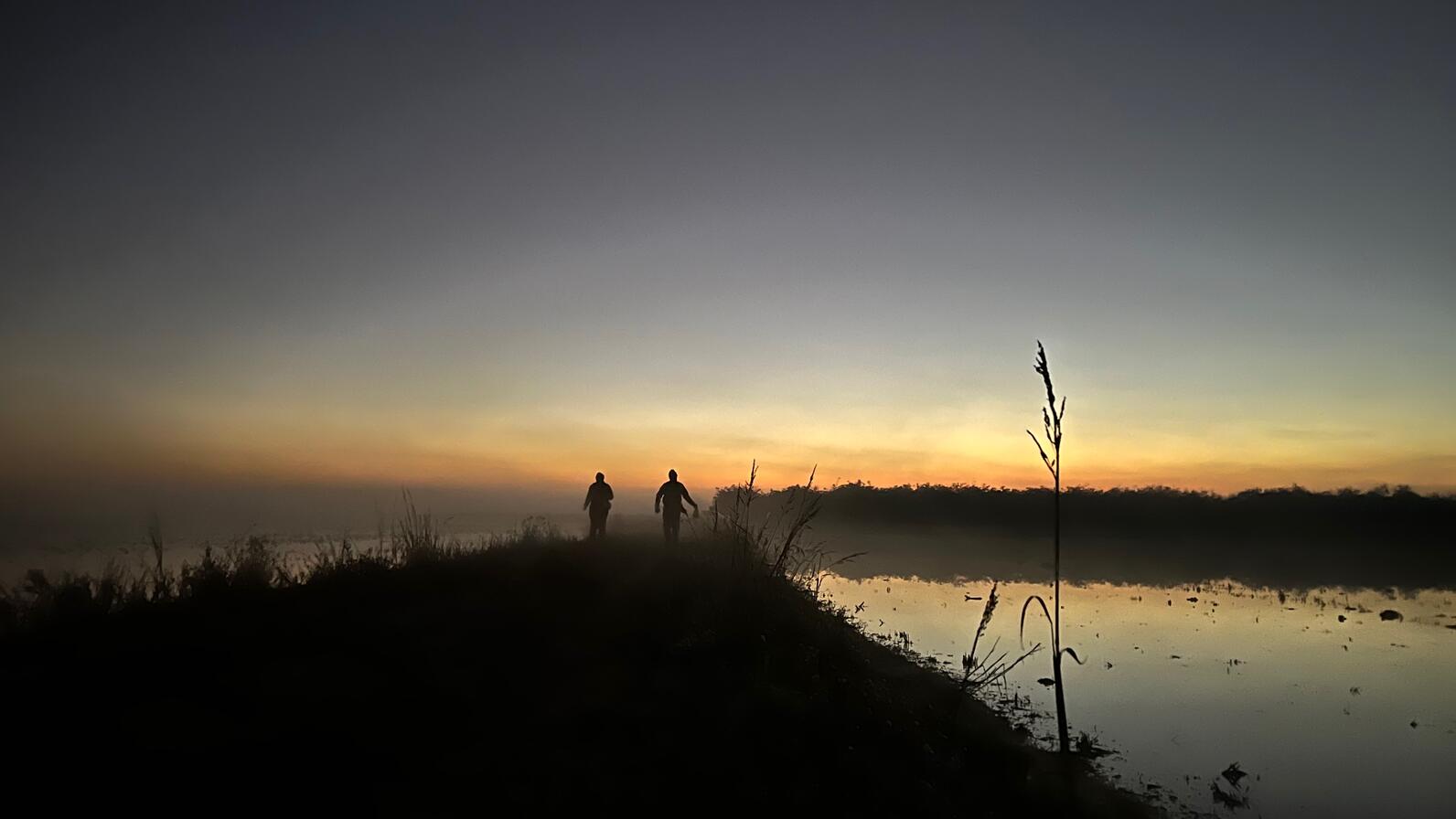In this evocative dusk scene, two men are seen walking into the distance along a narrow grassy path flanked by a marsh on either side. Their silhouettes are centered against the dramatic backdrop of a setting sun, which casts an orange and yellow hue at the horizon that transitions into a darker blue-grey sky, peppered with scattered, murky clouds. The men seem to be heading towards a distant forest of trees visible in the background. The water bodies on either side of the path reflect the vibrant colors of the sky, adding depth to the image. Cattails and various tall grasses delineate the edges of the path, creating a serene yet haunting atmosphere as day turns to night.